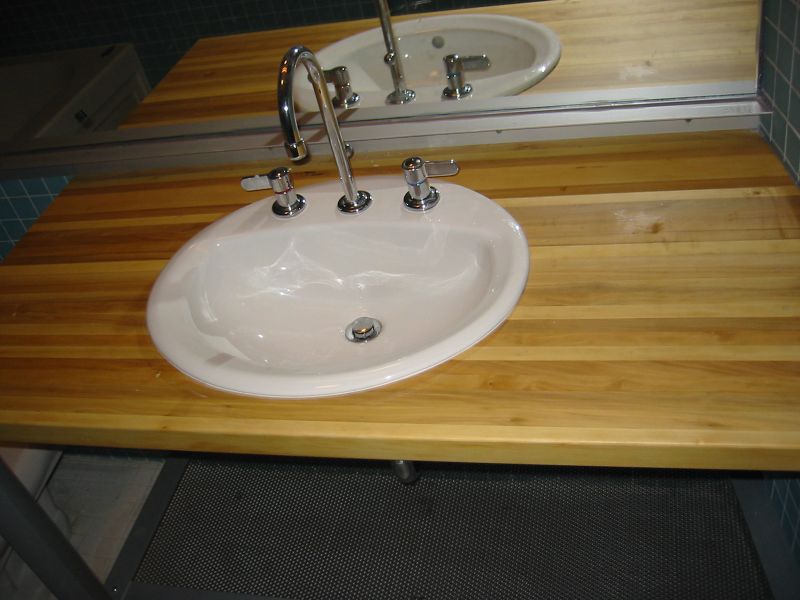The image features a uniquely designed countertop crafted from wood, displaying an elegant pattern of dark and white stripes. The countertop is adorned with a white porcelain sink, seamlessly inlaid, and accompanied by sleek silver hardware. Positioned above the countertop is a mirror, which reflects the sink, enhancing the room's spatial feel. Notably, the countertop lacks cabinets underneath, revealing its sturdy legs and the visible silver water pipe. The floor beneath showcases gray, brick-shaped tiles, accentuated by a subtle gray strip. Additionally, under the sink lies a lighter gray mat, exhibiting a tightly woven design reminiscent of a finely meshed screen, adding a distinctive texture to the space.